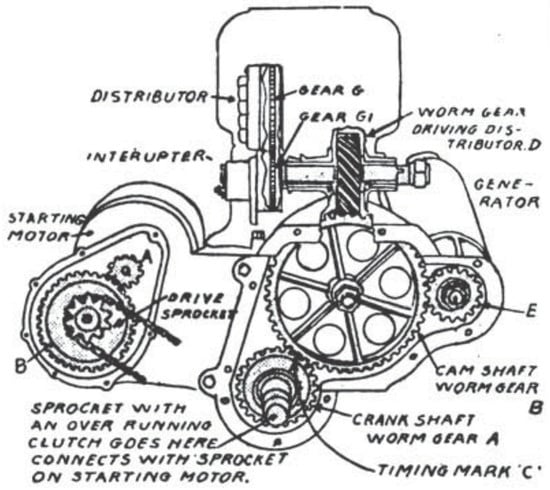This is a detailed black-and-white schematic drawing of a vehicle's engine, showcasing various interconnected components. At the top, the diagram labels the "Distributor" and "Interrupter," with pointers indicating their exact positions within the engine. Below, the labels "Gear G" and "Gear G1" denote specific gears in the assembly. A prominent "Starting Motor" is situated lower in the image, adjacent to a "Drive Sprocket." An instructive arrow indicates where a sprocket with an overrunning clutch connects to the sprocket on the starting motor, underlining its function and integration.

To the right, the schematic features the "Crankshaft" and "Worm Gear A," accompanied by "Timing Mark C," essential for accurate engine timing. The "Camshaft" is depicted above, linked with "Worm Gear B" and highlighted with the label "E" pointing to a disc-like component. This entire section is collectively referred to as the "Generator."

On the far right, the "Worm Gear Driving Distributor" is indicated, emphasizing its role within the intricate engine mechanism. The diagram thoroughly maps out the internal workings of the engine, from gears to sprockets, providing an instructional overview of the mechanical relationships and operations within.